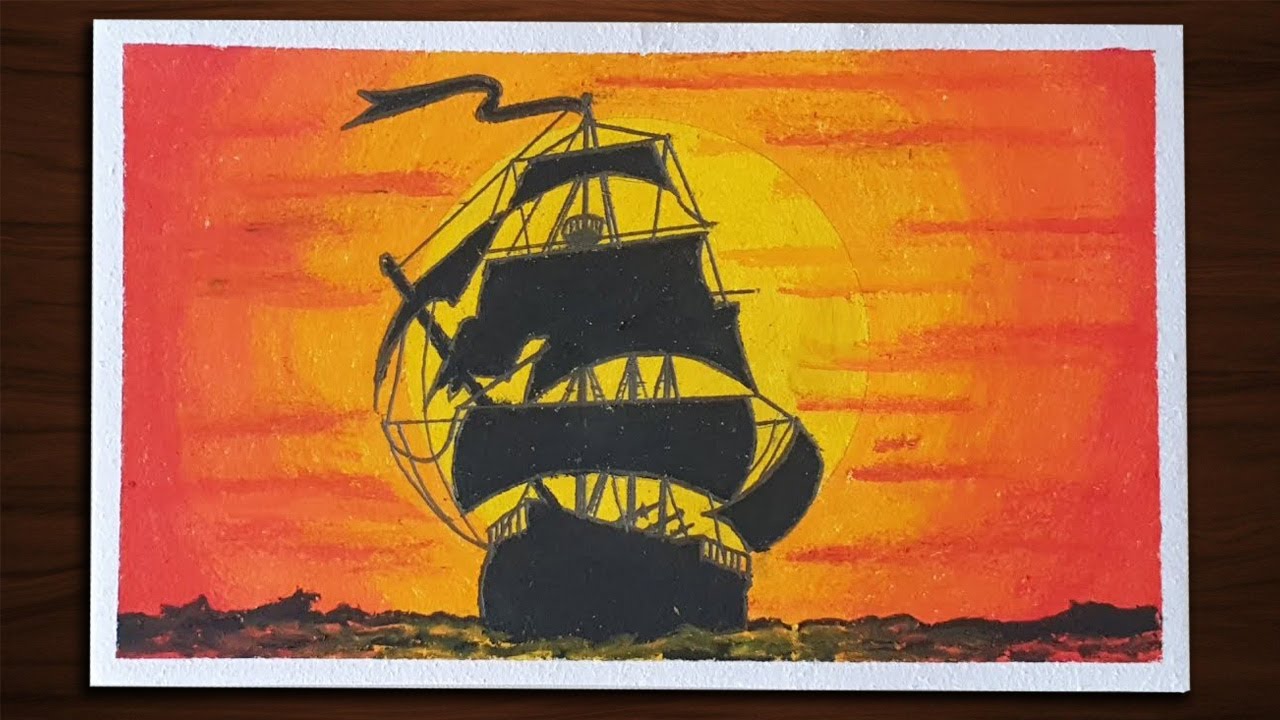This illustration depicts an old sailing ship, reminiscent of the 1400s, possibly from the Age of Sail, such as the Mayflower. The large vessel, which could be a merchant or pirate ship, is rendered with a detailed silhouette against a gigantic, setting or rising Sun that dominates the background. The black ship boasts multiple masts and fully deployed sails, indicating it is moving at full speed. A prominent long banner unfurls from the top mast, fluttering in the wind. The ship’s intricate design includes three levels of sails, a crow’s nest situated between the second and third levels, and visible details like railings, ladders, rigging, and three cannons on the deck. The sky around the Sun transitions from a bright yellow at the center, blending into deep orange and then red toward the edges. The dark, almost black sea below shows subtle movement, adding to the dynamic atmosphere of the scene. The painting appears to be crafted with acrylic or watercolor paint, given its grainy texture, and is bordered by a white frame, enhancing its classic and timeless appearance.